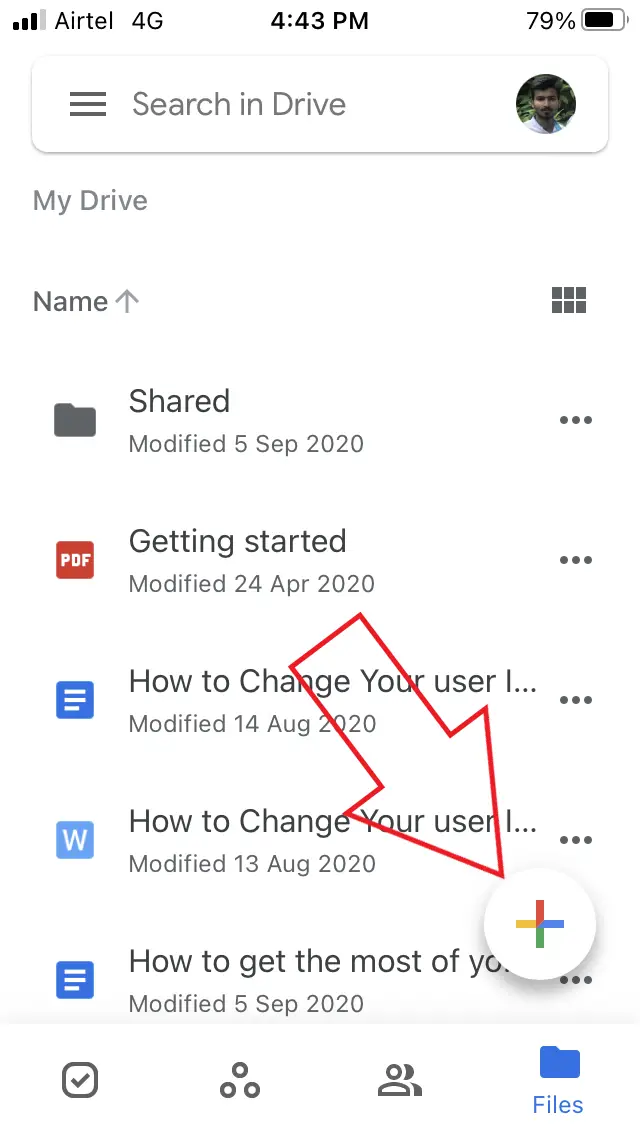The image is a screenshot from the Google Drive app interface. At the top, there's a prominent search bar labeled "Search in Drive." Below that, on the left side of the screen, it displays "My Drive." Additionally, towards the right, it shows the heading "Name" accompanied by an upward facing arrow, indicating a sorting option. Further down, there is a list of document titles which includes "Share," "Getting Started," "How to Change Your User," and a partially visible "How to Get the Most of Your..." with the remaining text obscured. Notably, the screenshot features a large red outline of an arrow pointing towards a multicolored plus sign encased within a white circle located at the bottom right corner of the screen.